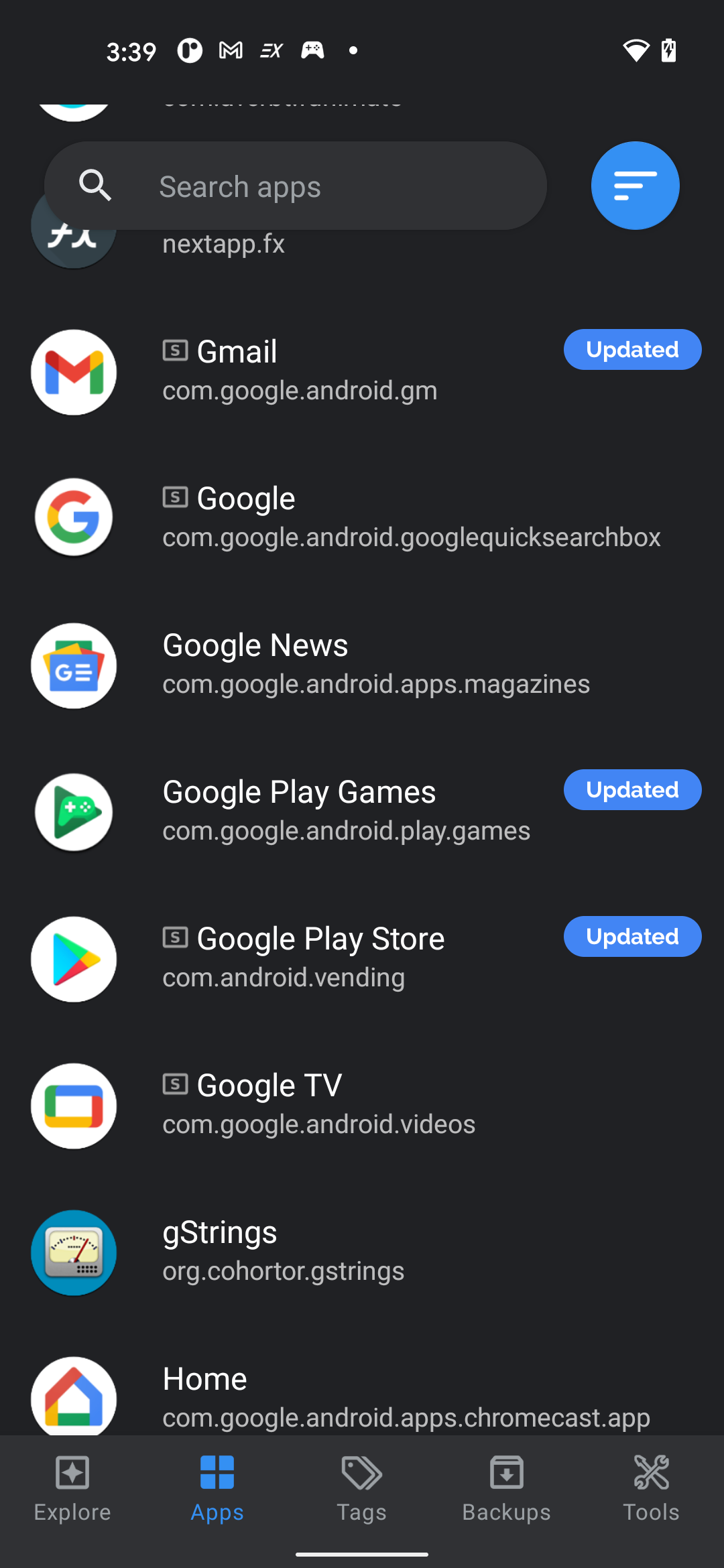A sleek digital display set against a black background shows a timestamp of 3:39. At the top, there's a prominent search bar featuring a magnifying glass icon on its left, indicating the function to search for apps. Below the search bar is a list of app shortcuts which include: Gmail, identified by the package name com.google.android.gm; Google Play Newsstand, referred to by com.google.android.apps.magazines; Google Play Games, listed under com.google.android.play.games; Google Play Store, recognized as com.android.vending; and Google TV, known by the package com.google.android.videos.